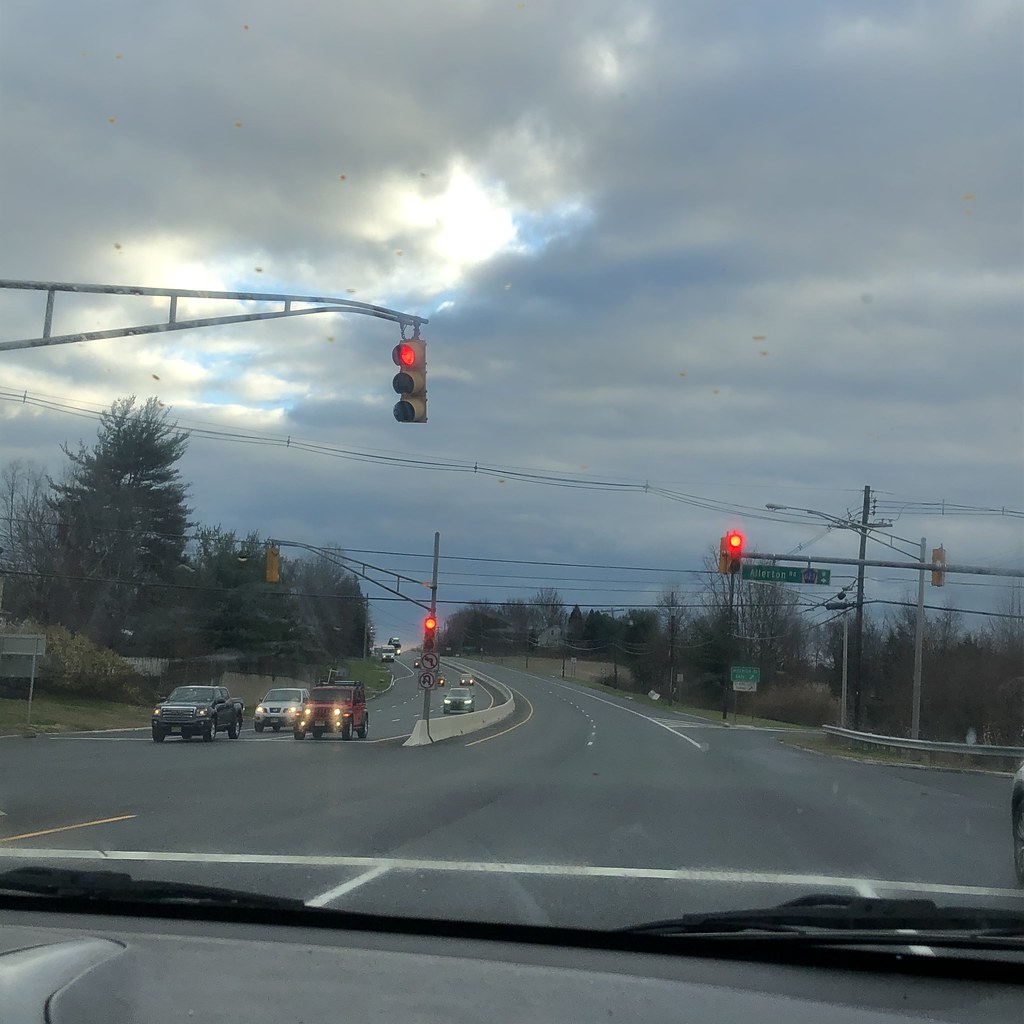In this image, taken from the front windshield of a car, we are looking at a bustling intersection at dusk. The sky is darkening, shrouded in dark clouds, with just a hint of blue remaining. In the foreground, the traffic light directly in front of us gleams red, halting the line of vehicles that extend into the distance. 

To our right, another road intersects, allowing vehicles to make left and right-hand turns, contributing to the dynamic flow of traffic. Prominently visible is a red Jeep positioned at the front of the left-hand lane, patiently waiting for the light to change. Behind it, a black truck and a variety of other cars continue to queue, their headlights illuminating the dimming evening.

On either side of the road, darkened trees frame the scene, while a cement barrier separates the outbound lanes from the oncoming traffic. Each road comprises two lanes, aesthetically mirrored by the dual-lane opposite heading towards and away from the intersection. The overall ambiance is marked by the interplay of artificial headlights against the encroaching night, encapsulating a moment of urban routine within a twilight setting.